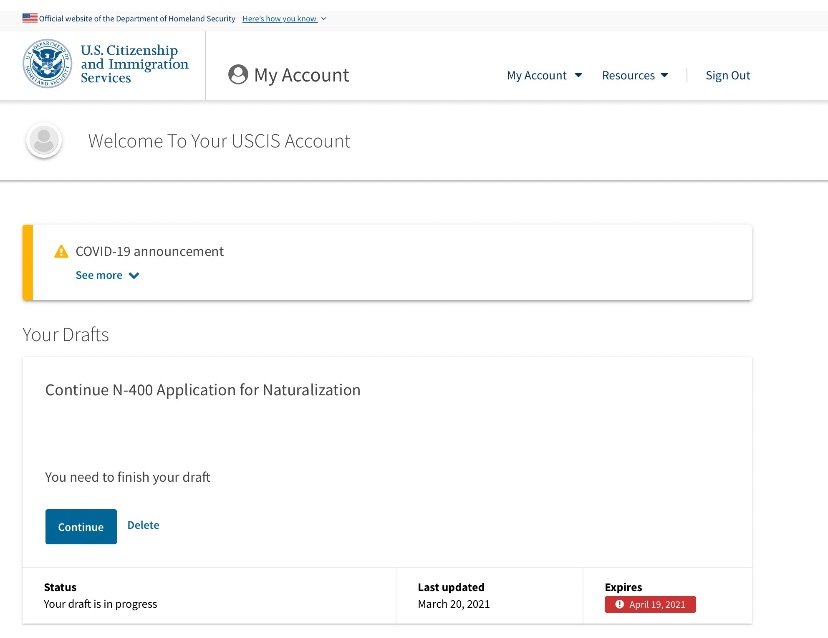The top section features a thin, light gray border with an American flag on the left. Adjacent to the flag, in blue text, it reads "Official website of the Department of Homeland Security." To the right, there is bright blue underlined text that says, "Here's how you know," accompanied by a gray downward-pointing arrowhead.

Beneath this, on a white background, the left side displays the United States seal, a very official-looking logo. To the right, in blue font, it reads "U.S. Citizenship and Immigration Services." A gray line serves as a divider below this text. To the far right, there's a traditional circular icon with a gray background, featuring a silhouette of a head and body, indicating the user's account. Next to this, in gray text, it says "My Account," followed by the same text in blue and a filled blue downward-pointing arrowhead, indicating a dropdown menu. Adjacent to this, it says "Resources," also with a downward-pointing arrowhead. Next to this is a small gray dividing line, then the blue text "Sign Out."

Another gray, shadowed border encases the user symbol on the left again, but this time it has a white border around it. To the right, in gray text, it says, "Welcome to your U.S.C.I.S. account," with only the "A" in "account" capitalized. Below this, another gray, shadowed border is present.

A notification follows, identifiable by its rectangular shape and white background. To the left of this rectangle, a bold strip of orange is visible. To the right, there is an orange triangle with a white exclamation point inside, indicating a warning.